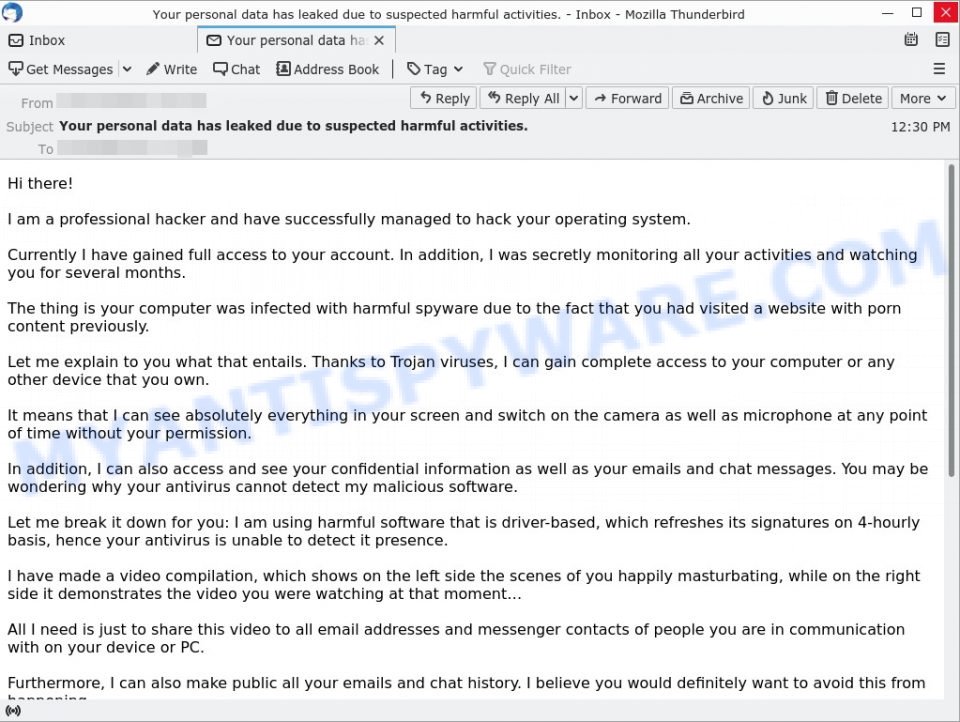The image depicts the interface of an email client, Mozilla Thunderbird, displaying a potentially alarming message about a data breach. At the top, a horizontal white bar spans the width of the page, featuring a blue symbol on the top left. Centered within this bar is a bold notification: "Your personal data has leaked due to suspected harmful activities." To the top right are the standard minimize, maximize, and close buttons, with the close button marked by a distinctive red "X."

Directly beneath this bar, the email client's main interface is visible. On the left side, a sidebar shows various tabs, with the "Inbox" tab highlighted, indicating it's currently in view. Within the main window, an email alert is open, reiterating that "Your personal data has leaked due to suspected harmful activities." Both the "From" and "To" lines of the email are intentionally blurred to maintain privacy.

The email's subject line mirrors the notification, repeating the concerning message about the data breach. Following the subject, there is a substantial block of text detailing the suspicious activities that led to the data leak. In the background, a watermark-like text, "myantispyware.com," is faintly visible in blue, suggesting a source or a tool related to the security issue.